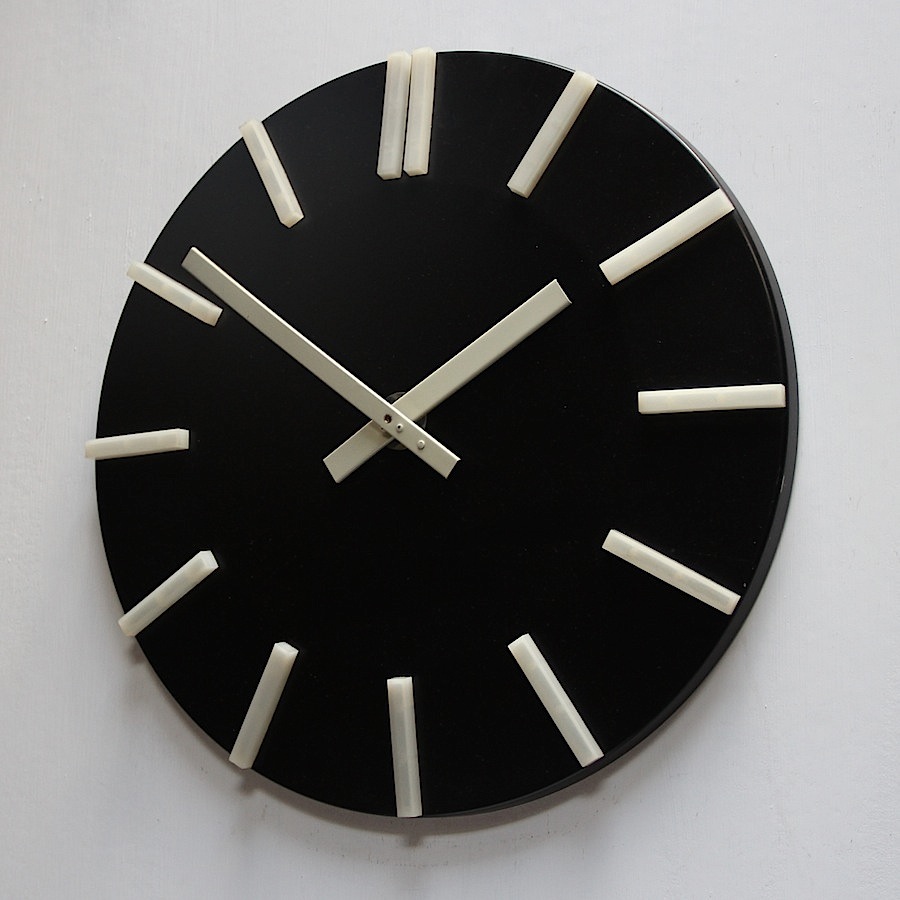This close-up photograph captures a modern clock affixed to a stark white wall. The clock is a sleek, minimalist design—essentially a flat, black disc without a frame. Instead of traditional numbers, the clock features white bars to indicate each hour, with every hour marked by a single bar except for the 12 o'clock position, which is denoted by two parallel bars. The clock hands are made of a white, metal material and are rectangular in shape, contrasting sharply against the black face. These hands are secured by a central silver circle, fastened with two or three screws. The time on the clock reads 1:52, as evidenced by the positions of the hour and minute hands. The background remains pristine and unadorned, emphasizing the simplicity of the clock while the minimalist design is further highlighted by a subtle shadow cast beneath the clock on the wall.